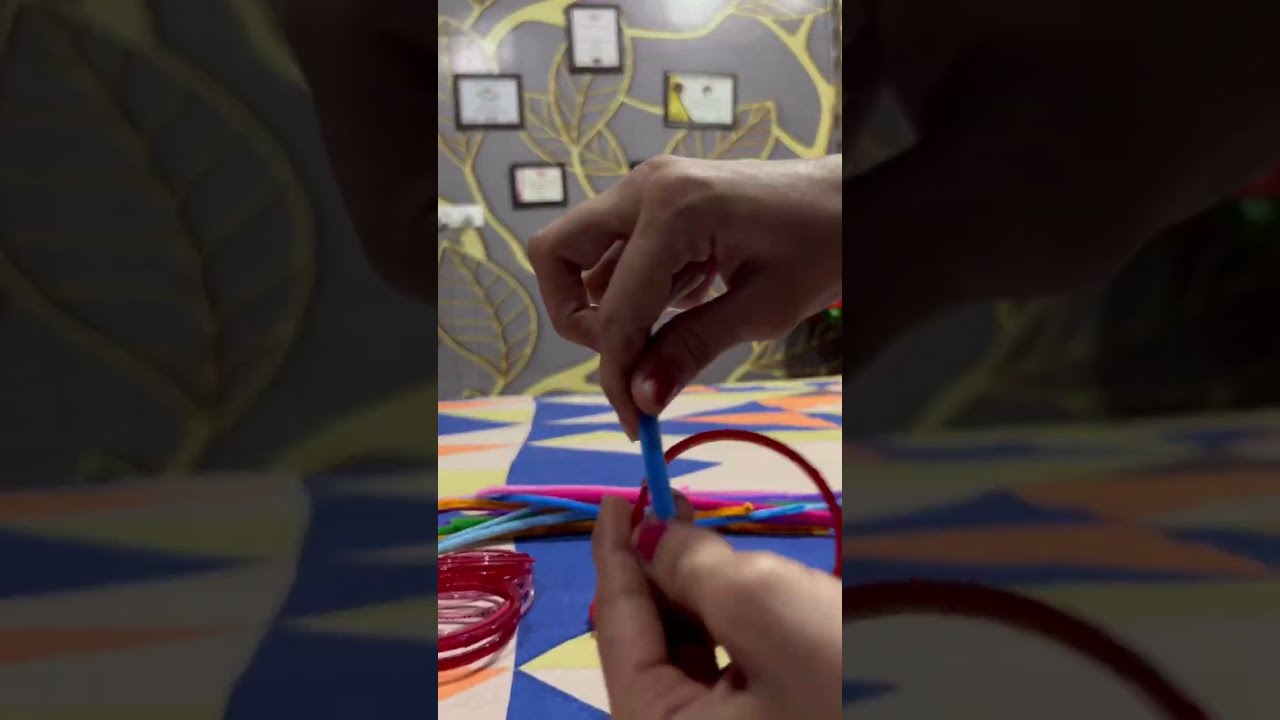This photograph captures a person engaged in a craft activity at a table, wrapped in a vibrant, geometric-patterned tablecloth featuring interlocking blue, orange, white, and yellow triangles. The individual’s hands, adorned with dark pink nail polish, are prominently displayed as they manipulate a blue plastic tube and a red plastic loop, which resemble thick, colorful spaghetti-like wires. The setting includes a gray wall decorated with an elegant gold leaf vine motif, and four discreet picture frames lining the background. The image appears layered, giving a sense of depth with the main, upright photograph in the center and two additional, darker and wider, repeated images behind it, creating a visually striking composition.